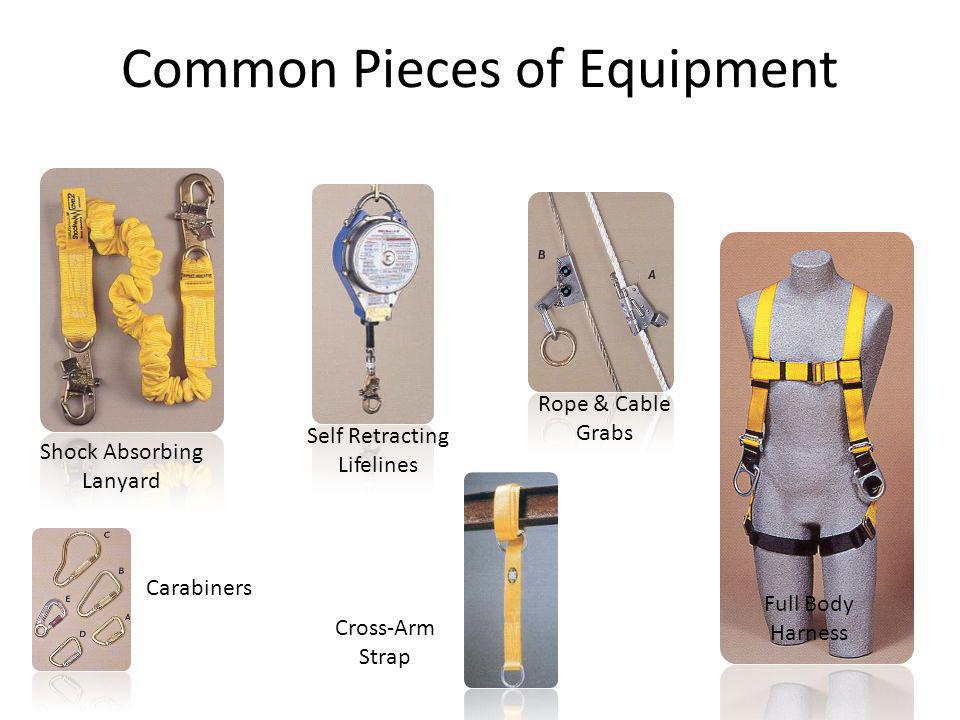The image is an infographic displaying various common pieces of equipment used for climbing, with a clean white background. The title "Common Pieces of Equipment" is prominently displayed at the top in black text. There are six detailed images of different equipment types, each within its own rectangular box featuring beige and dark brown backgrounds, along with descriptive black text labels.

Starting from the top left, the first image shows a yellow-colored shock absorbing lanyard, scrunched in the center, with bronze-colored clips on both ends. Moving to the right, the next image is of a self-retracting lifeline, resembling a round metal drum with a line extending from its bottom. The third image on the top row displays rope and cable grabs, illustrated as thin metal cables.

On the bottom row, starting from the left, the first image showcases various carabiners labeled A, B, C, D, and E in different sizes. The next image in the middle is of cross arm straps, which are yellow belts with rings or hooks on both ends. The final and largest image to the far right features a yellow full body harness displayed on a gray mannequin without a head or arms. Each piece of gear is meticulously labeled and illustrated, suggesting they are essential tools for climbing activities.